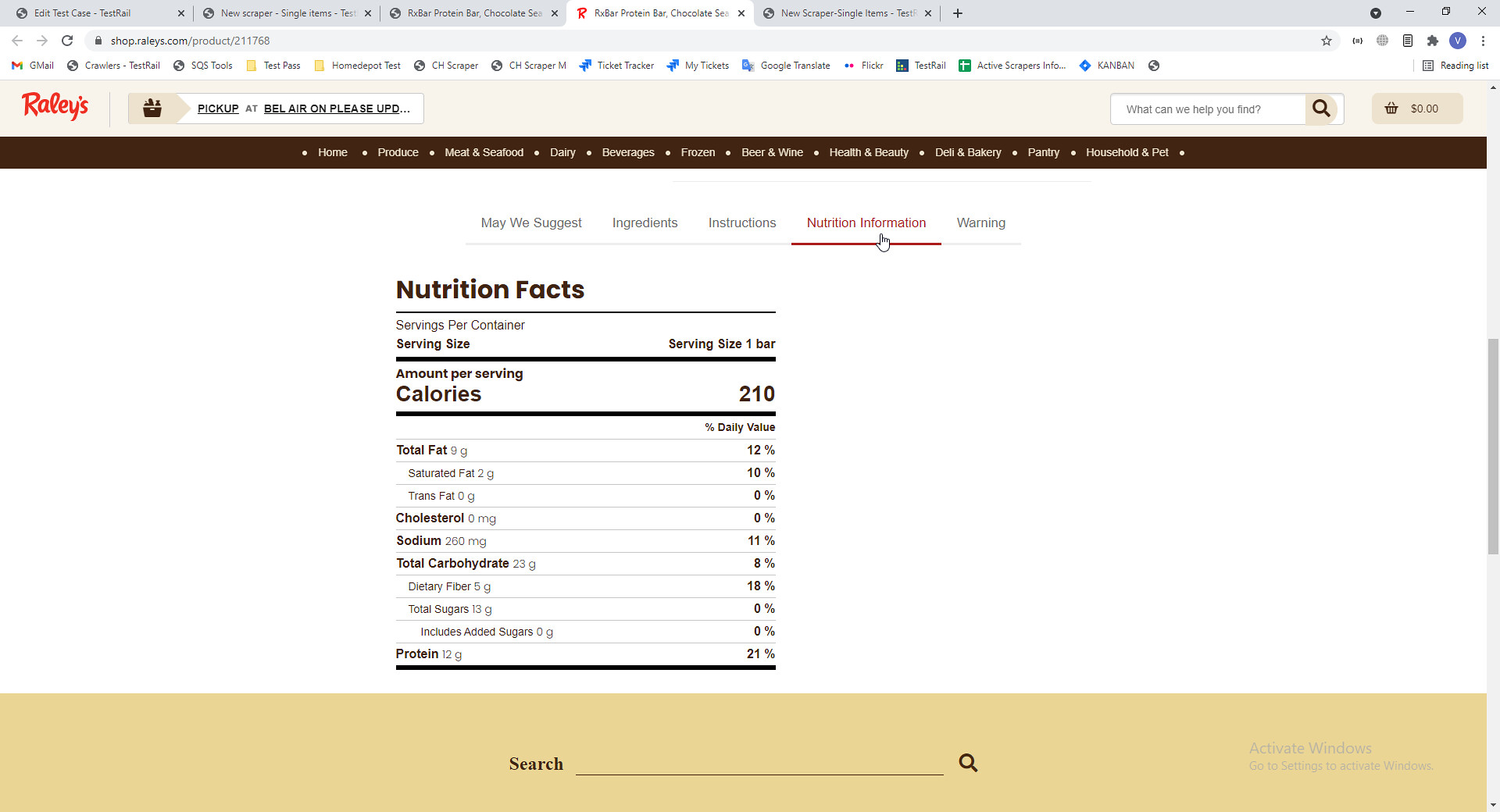The image shows a computer screen with a centrally displayed webpage featuring a nutrition label. The nutrition label is prominently visible, providing detailed nutritional information. The browser has five open tabs, listed from left to right as follows: "May We Suggest," "Ingredient Instruction," "Nutrition Information," and "Warning." 

Beneath the heading "Nutrition Facts," the label specifies several key details:
- "Serving Per Customer."
- "Serving Size," indicated as "Serving Size 1 Bar."
- "Amount Per Serving," detailing the various nutritional values.

Highlighted nutritional information includes:
- "Calories: 210."
- "Total Fat: 9g, which represents 12% of the Percent Daily Value."
- "Saturated Fat," with unspecified amounts and daily values due to the cutoff.

The neatly organized layout and clear presentation of nutritional data make it easy for users to understand the dietary content of the product.